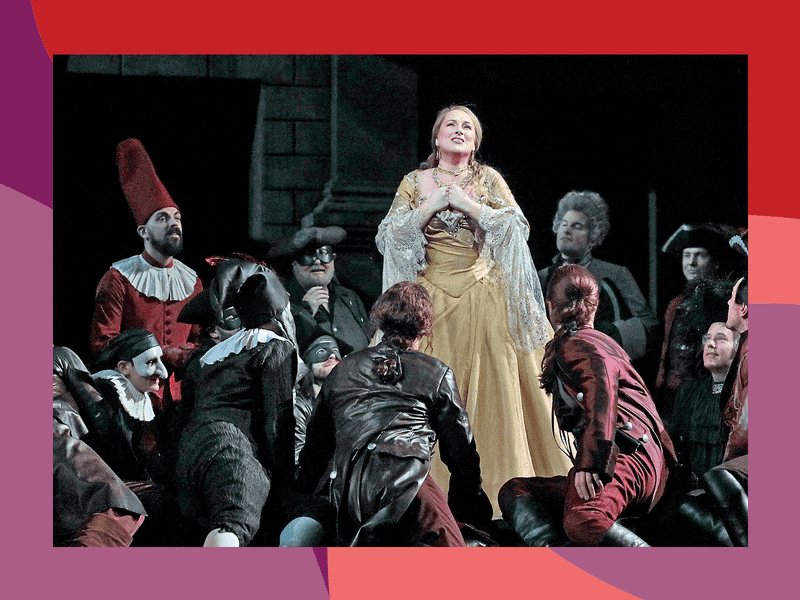The photograph is a detailed live shot of a scene from a Shakespearean play, set on a stage with a brick wall backdrop. Dominating the right center of the image is a woman in period attire, reminiscent of the 19th century. She has long blonde hair pulled back and is adorned in a beige or gold ball gown with white lacy sleeves, clasping her hands together as she either sings or delivers a monologue, looking upward towards the audience. Surrounding her are male cast members, arranged in various positions—some sitting, some standing, and others partially reclining. A variety of colorful costumes enrich the scene: a man in a maroon outfit with a large pleated white collar and tall dunce cap, a clown wearing a black coat and a mask with an elongated nose, and other men clad in burgundy and black leather waistcoats, maroon hats, and black boots. Soldiers in British pointed caps and cloaks stand in the right foreground. The scene is framed by an artistic border of red, light purple, and light orange hues. The palette of the entire composition includes black, maroon, beige, white, and yellow, creating a vivid and dynamic tableau.